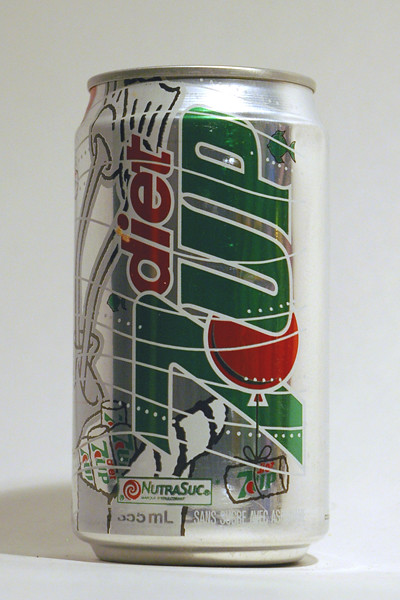The image showcases a can of diet 7-Up soda. The can is primarily silver, with a slightly lighter shade of silver covering the main body compared to the more reflective aluminum of the top ridge and lid area. The iconic 7-Up branding is featured prominently, with "7-Up" written in large green letters outlined in white, and a small red round ball situated between the "7" and the "U." Above the main logo, the word "diet" is displayed in red letters, also outlined in white. Near the bottom of the can, a white box contains the text "Nutri-Suck," which likely denotes some type of artificial sweetener, alongside a small red flower icon. The can is placed on a light-colored surface with a similarly light background, emphasizing the sleek and reflective qualities of the can.